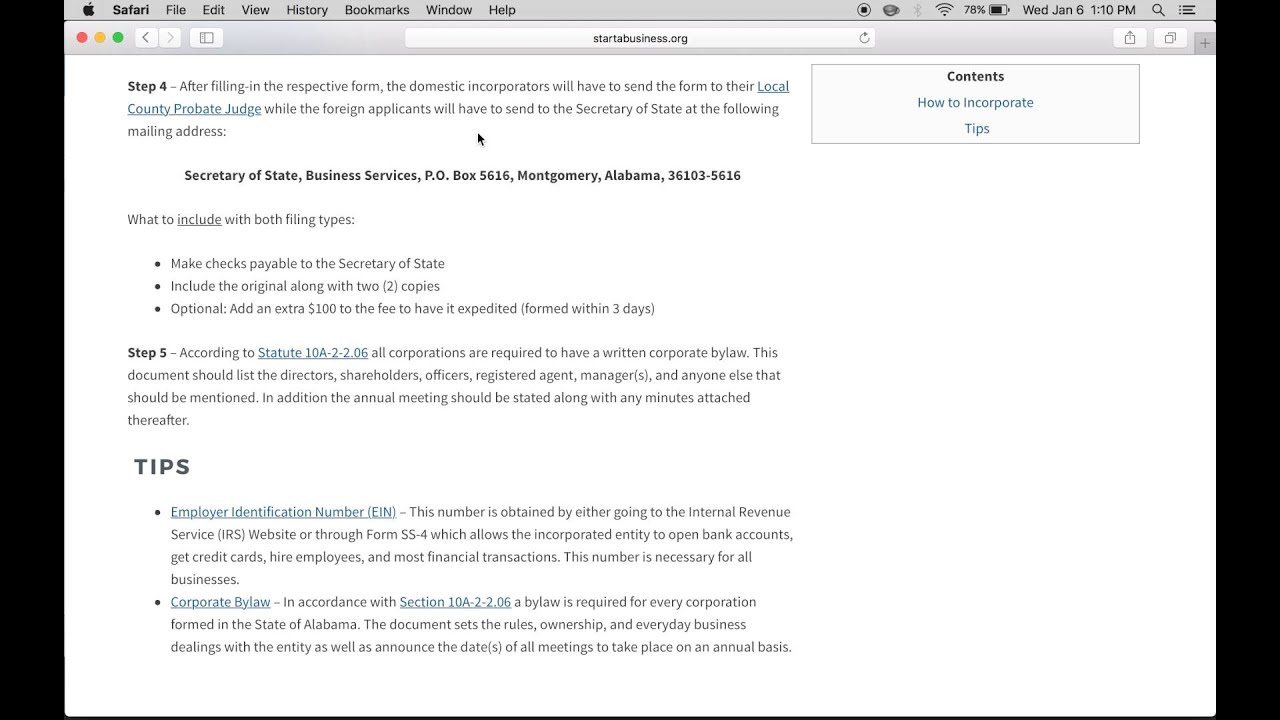This image is a screenshot of a web browser window in Safari, showcasing a webpage with step-by-step instructions. The screenshot features black borders on both the left and right sides. 

At the top of the window, the Apple logo is visible in the upper left corner, followed by "Safari" and the menu options: File, Edit, View, History, Bookmarks, Window, and Help. On the right side of the top bar, various system icons are displayed, including battery status, the date and time (Wednesday, January 6th, 1:10 p.m.), and a search button.

Below the top bar, on the left-hand side, there are three colored circles (red, yellow, and green) that are typical for window control buttons in macOS, along with back and forward navigation arrows. Centrally located beneath these features is the address bar, which appears to be empty or not prominently showing a URL.

The main content of the webpage below the address bar has a white background. Visible on this page is a section labeled "Step 4," followed by the text "Secretary of State Business Services, P.O. Box 5616," indicating instructions related to the Secretary of State’s office in Montgomery, Alabama. At the bottom of the page, there is a section marked "Tip," providing additional information or guidance.

Overall, the environment suggests that the user is navigating through a form or set of instructions on an official website.